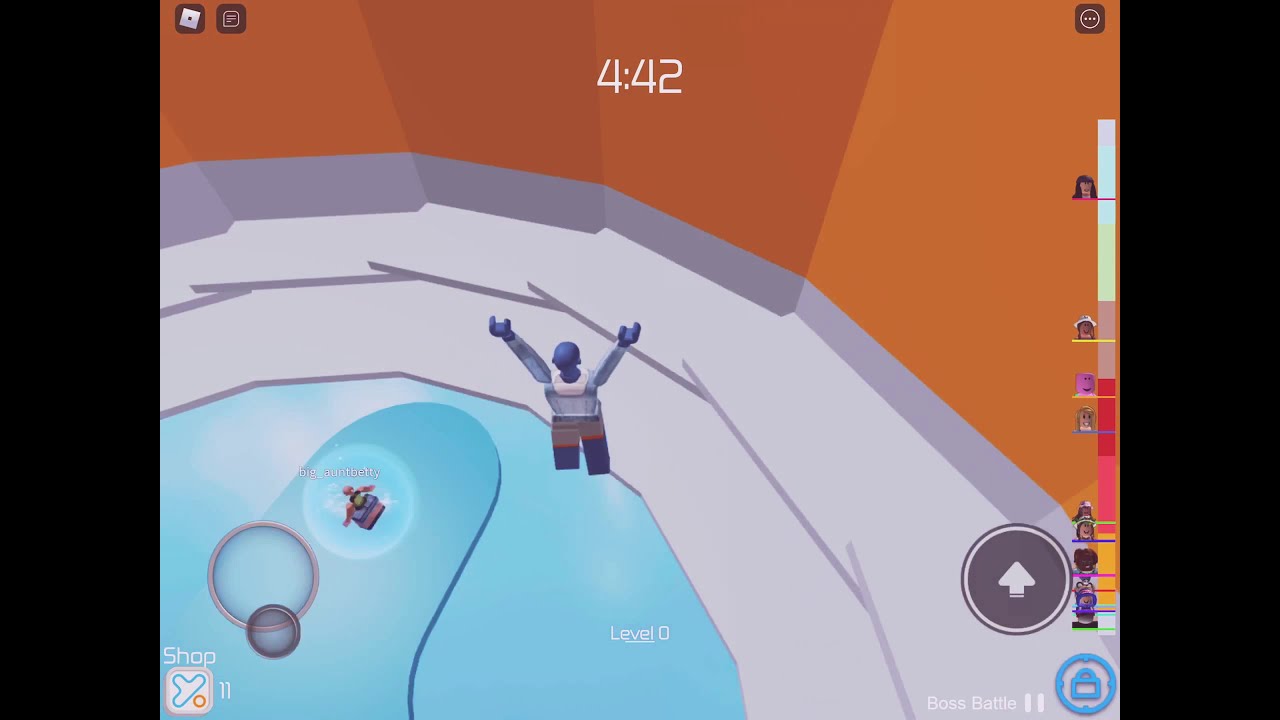The image is a detailed screenshot from a video game, likely Roblox. It features a blocky, robotic-looking character with blue arms, hands, head, and neck, resembling a LEGO figure. The character stands with its arms raised in an environment that includes orange and gray walls, a light blue floor, and a light gray floor. The background shows complex game elements such as an "upload" button (a circular icon with a white upward-facing arrow) and a "boss battle" text with a pause button located at the bottom right. The right side of the screen displays a meter featuring colorful sections (white, yellow, pink, red, gray, green, and blue) alongside multicolored lines and icons of people. Above, a timer reads "4:42." The surrounding area includes a gray circular sidewalk and some water, all within an orange and gray wall enclosure, and the username of another player is visible.